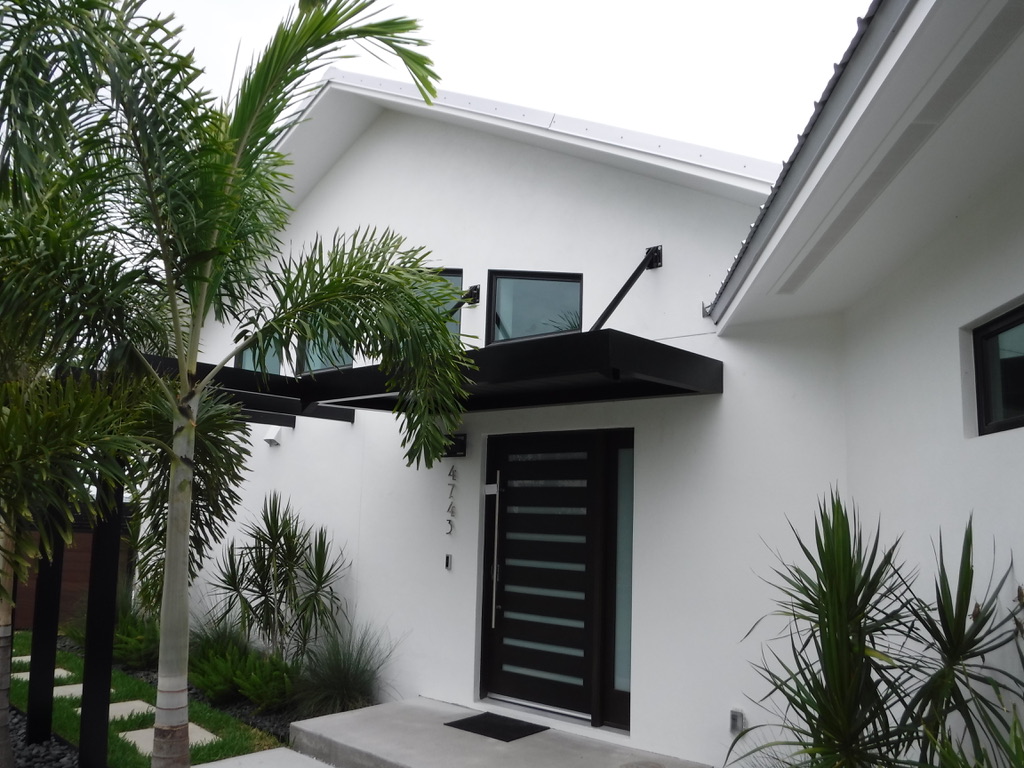This image captures the entrance of a modern-styled house, characterized by its clean white stone walls and sleek design elements. Centrally positioned, the black door stands out with its horizontal gray lines and long silver handle. Directly above the door, there are four square-shaped windows of varying lengths. The house number "4743" is prominently displayed to the upper left of the door. 

The front porch, slightly offset to the side, features a black overhang supported by metal braces. Below, a cement block entryway and steps lead up to the door. Multiple palm trees and other greenery embellish the scene, with one prominently positioned in the lower left corner and another on the left side of the photo, adding a touch of natural beauty to the modern facade. The triangular roof is visible at the very top, along with a clear white sky, framing the entire view in a serene yet sophisticated manner.